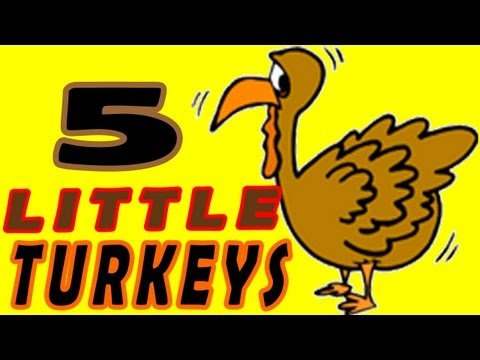The image features a digitally-rendered turkey set against a solid yellow rectangular background, bordered by thick black rectangles at the top and bottom. The turkey, depicted in brown with lines illustrating its feathers, small orange feet, and an orange beak and wattle, is positioned on the right side of the image. It faces left towards the text and has an eye looking towards the viewer, giving it a sad or nervous expression. Surrounding the turkey's beak, head, and body are lines indicating a slight trembling.

To the left of the turkey, there is a large black number "5" with a thick light brown outline. Beneath the "5" is the word "LITTLE," written in dark brown capitals outlined in red, followed by the word "TURKEYS" in black capitals outlined in orange. Both words are stacked one above the other. The text and the image are centrally aligned within the bordered yellow section, creating a clean and balanced composition that suggests a digital design, potentially for a meme or a digital presentation.